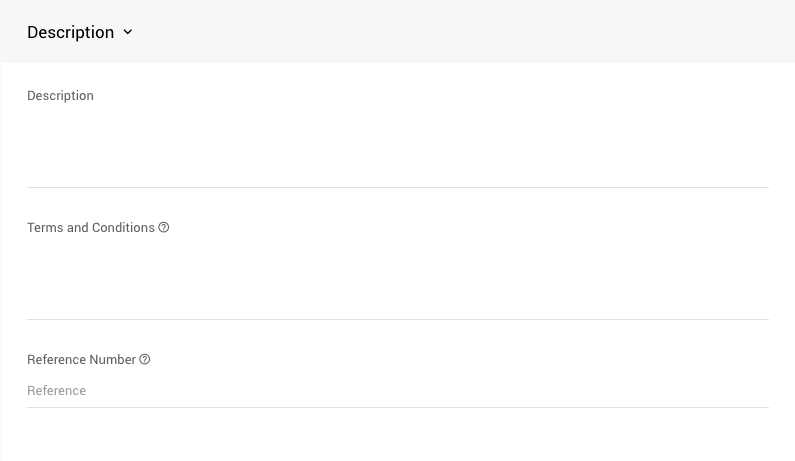**Website Page Overview**

The webpage features minimal content and employs a predominantly gray color scheme. At the top of the page, a black text description is displayed within a gray bar, providing a brief overview. Below this bar, a drop-down menu offers various selectable options for user interaction.

Following this, the word "Description" appears again in gray letters, with a gray line beneath it separating the sections. The next section lists "Terms and Conditions" in gray letters, accompanied by a small question mark icon within a circle for additional information.

Subsequent to this, another gray line introduces a section labeled "Reference Number," also in gray letters, with a corresponding question mark icon in a circle for more details. Directly beneath, the page repeats the term "Reference" in gray letters.

The page is notably sparse with no further content or branding, offering no indication of the website's purpose or the company associated with it. The repetitive and minimalist design leaves little room for additional description.